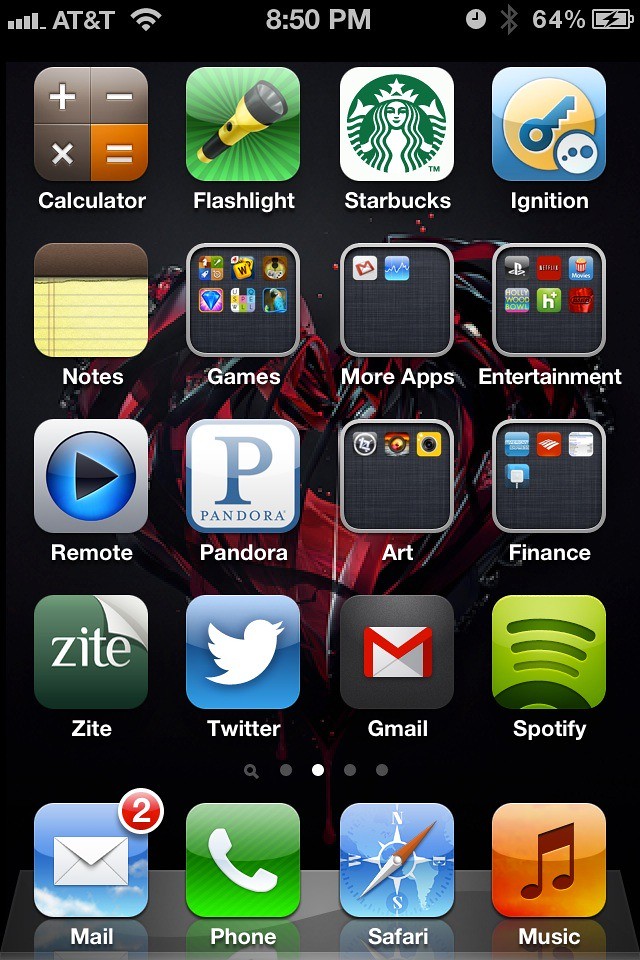This photo captures someone's meticulously organized smartphone home screen. The layout features five rows and four columns of various apps and folders against a black background accented with a striking red artistic design in the center.

- **Top Row**: From left to right, the apps are Calculator, Flashlight, Starbucks, and Ignition.
- **Second Row**: The layout includes a Notes app on the far left. Following it is a black folder containing six apps arranged in a 3x2 grid, another black folder with two apps side by side, and a folder named Entertainment which holds six apps, also in a 3x2 configuration.
- **Third Row**: This row starts with the Remote app on the left, followed by Pandora. Next is an Art folder housing three apps and a Finance folder containing four apps.
- **Fourth Row**: The apps here are Zeit, Twitter, Gmail, and Spotify.
- **Bottom Row (Dock)**: There's a Mail app featuring a small red circle with the number "2" indicating unread messages, flanked by Phone, Safari, and Music apps.

The overall aesthetic is clean yet vibrant, thanks to the distinctive red design that contrasts with the dark backdrop.